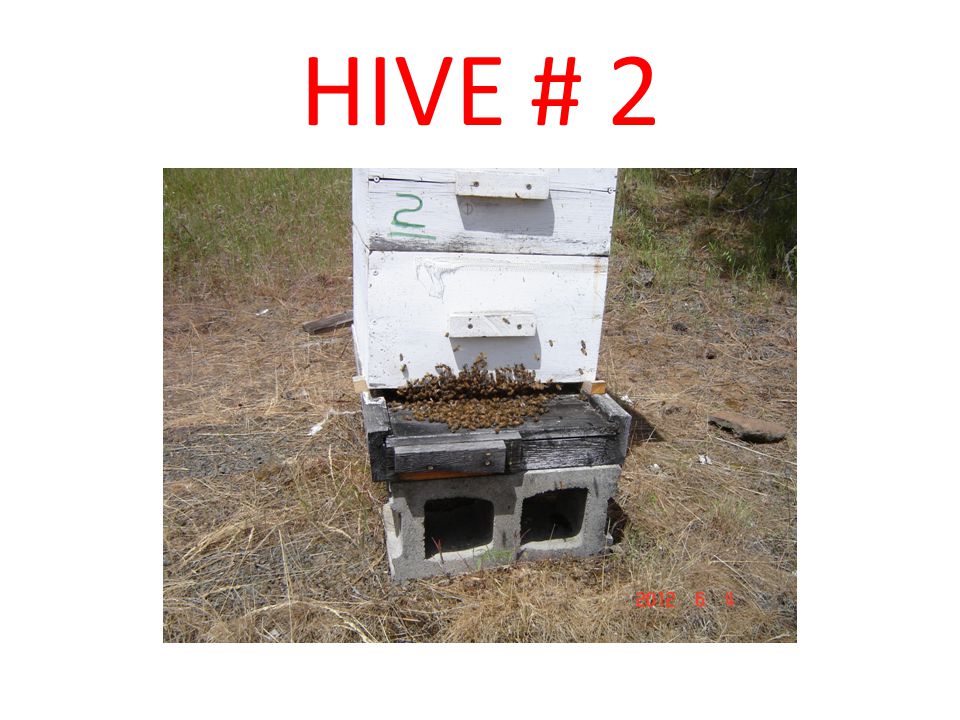This outdoor photograph depicts a beehive labeled "HIVE #2" in red capital letters at the top. The hive is constructed on a somewhat weathered setup that begins with a gray concrete slab featuring two prominent holes. Above this slab sits a dark wooden plank where numerous bees are visible. This wooden plank supports two white-painted wooden containers, one stacked on top of the other, with bees emerging from the gap between these containers and the plank below. The surrounding ground is covered in patches of green and brown grass, with areas of dirt and dead grass evident. In the bottom right corner, the date "2012 6 8" is inscribed.